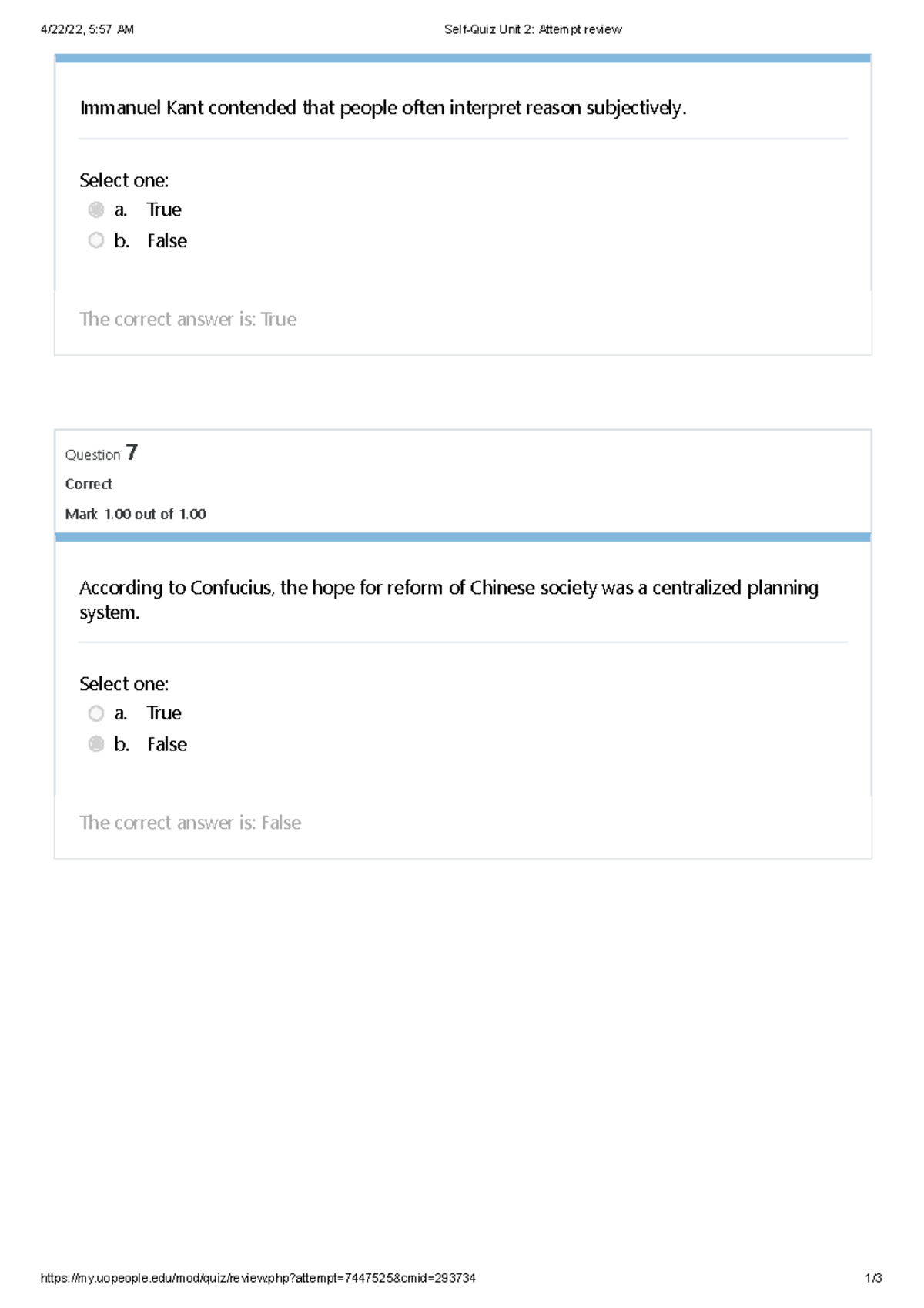A detailed screenshot of an online test for a philosophy class, dated April 22, 2022, at 5:57 AM, captures the user’s attempt review for "Self-Quiz Unit 2." The screen prominently features two graded questions in large gray boxes with white backgrounds. The first question states, "Immanuel Kant contended that people often interpret reasons subjectively," with answer options "true" or "false." The user selected "true," which is encircled and accompanied by the confirmation in light gray text, "The correct answer is true." The second question, labeled "Question 7," asks, "According to Confucius, the hope for reform of Chinese society was a centralized planning system," again with "true" and "false" options. The user selected "false," which is also circled and verified by the text, "The correct answer is false." Both answers are correct, as indicated by the grading annotations.